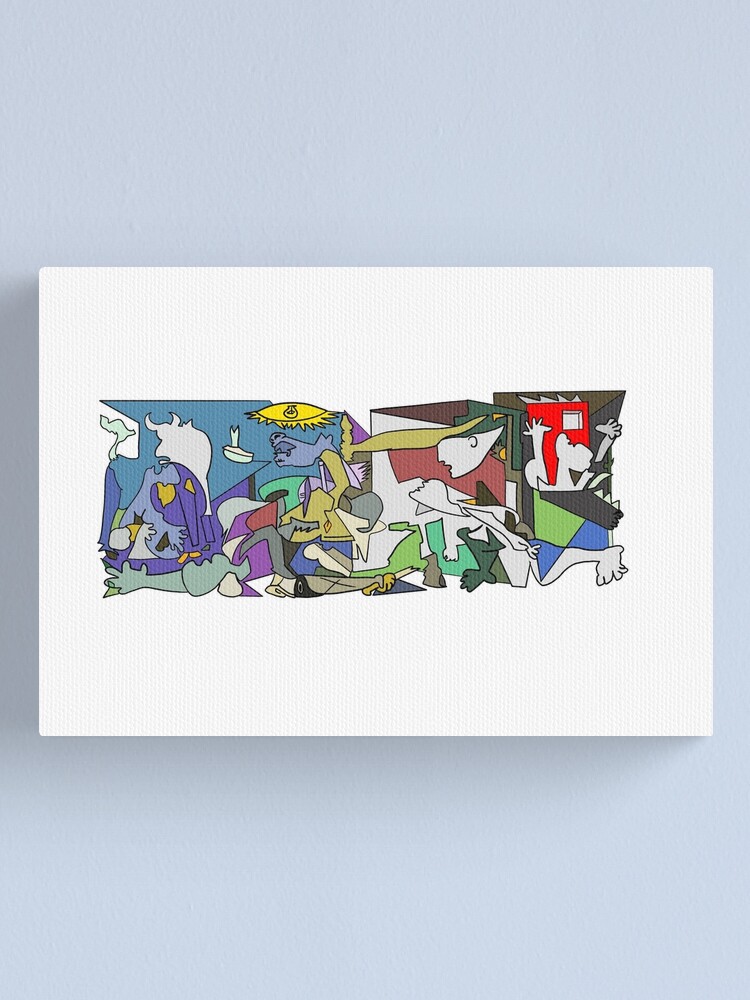This image is an abstract, surrealistic painting reminiscent of the styles of Picasso or Dali, featuring a plethora of colors including blue, yellow, green, red, purple, and aqua. It is set within a rectangular frame with a light blue background, centered on a lighter blue square. The painting is brimming with chaotic and vibrant elements. On the left, there appears to be a headless figure or just a t-shirt without a head, surrounded by hues of purple and yellow. Nearby, a very blue man dressed in a yellow t-shirt is depicted walking. The scene also includes a yellow, UFO-like shape at the top, adding to the eccentricity. Toward the center, there is chaos with various abstract figures; one figure lies flat on his stomach reaching out, while another figure, located on the right, seems to be on his knees attempting to go through a red door with a small window. Additionally, there are floating heads and the outlines of animals mixed into the composition. Near the red door, a man is seen with his hands raised, next to what seems to be a red book. The painting masterfully blends these elements with a wild mix of colors, creating a captivating, dreamlike scene.